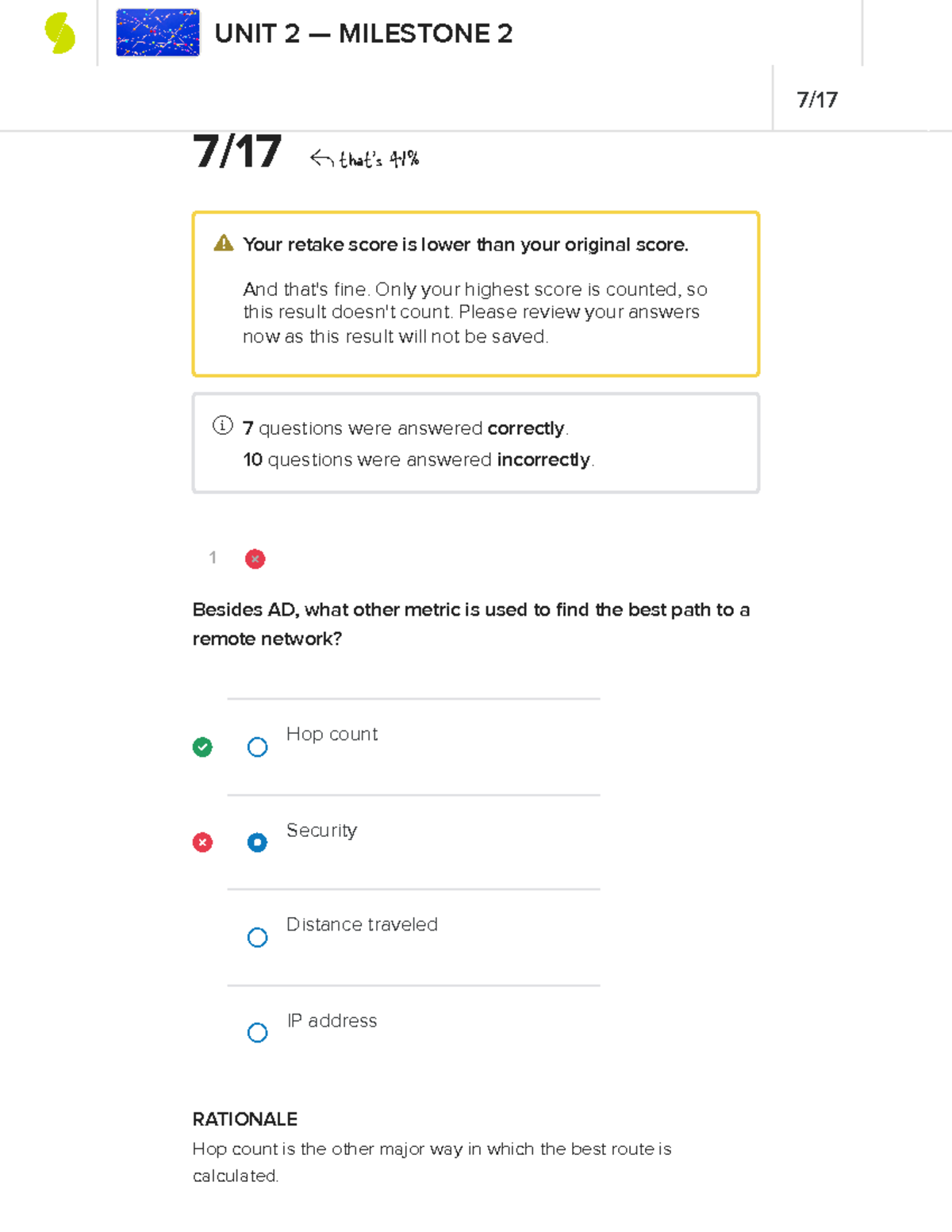In the upper left corner of the image, there is a small blue square. Next to this square, in black text, it reads "Unit 2 - Milestone 2." Moving to the right, the numbers "7-17" are repeated twice. A tiny green circle also appears in the upper left corner, with an arrow pointing to "7-17" and indicating "41%."

Below this, within a square, there is a message stating: "Your retake score is lower than your original score, and that's fine. Only your highest score is counted, so this result doesn't count. Please review your answers now as this result will not be saved." 

Another smaller square informs that "Seven questions were answered correctly. Ten questions were answered incorrectly."

A small red circle features a question: "Besides AD, what other metric is used to find the best path to a remote network?" This is followed by multiple options: 
- A tiny green circle with a check mark next to the correct answer, "Hop count."
- A blue circle with the word "Security."
- The words "Distance traveled" and "IP address."

At the bottom, there is a rationale: "Hop count is the other major way in which the best route is calculated."